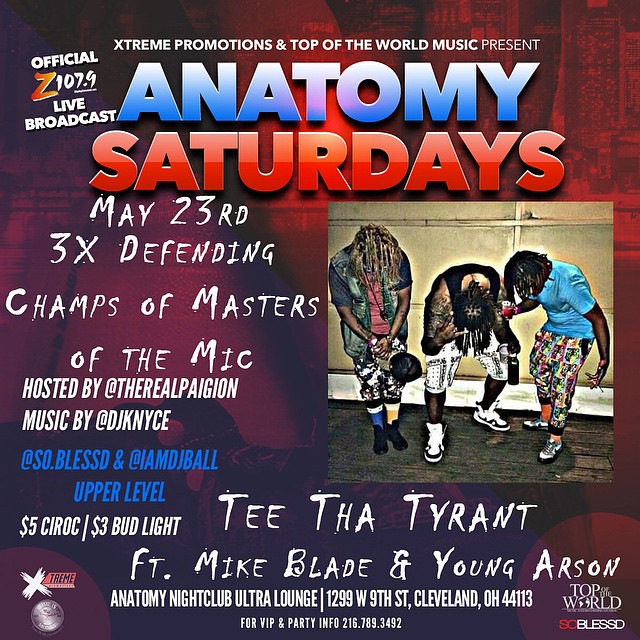Promotional flyer for the "Anatomy Saturdays" event at Anatomy Nightclub Ultra Lounge, located at 1299 West 9th Street, Cleveland, OH 44113, on May 23rd. The event is presented by Extreme Promotions and Top of the World Music, featuring an official live broadcast by Z 107.9. Headlining the night will be the 3x defending champs of 'Masters of the Mic,' hosted by @TheRealPygyon, with music provided by @DJKints. Special performances by Tita Tyrant featuring Mike Blade and Young Arson. Drink specials include $5 Serac and $3 Bud Light. For VIP and party info, contact 216-789-3492.